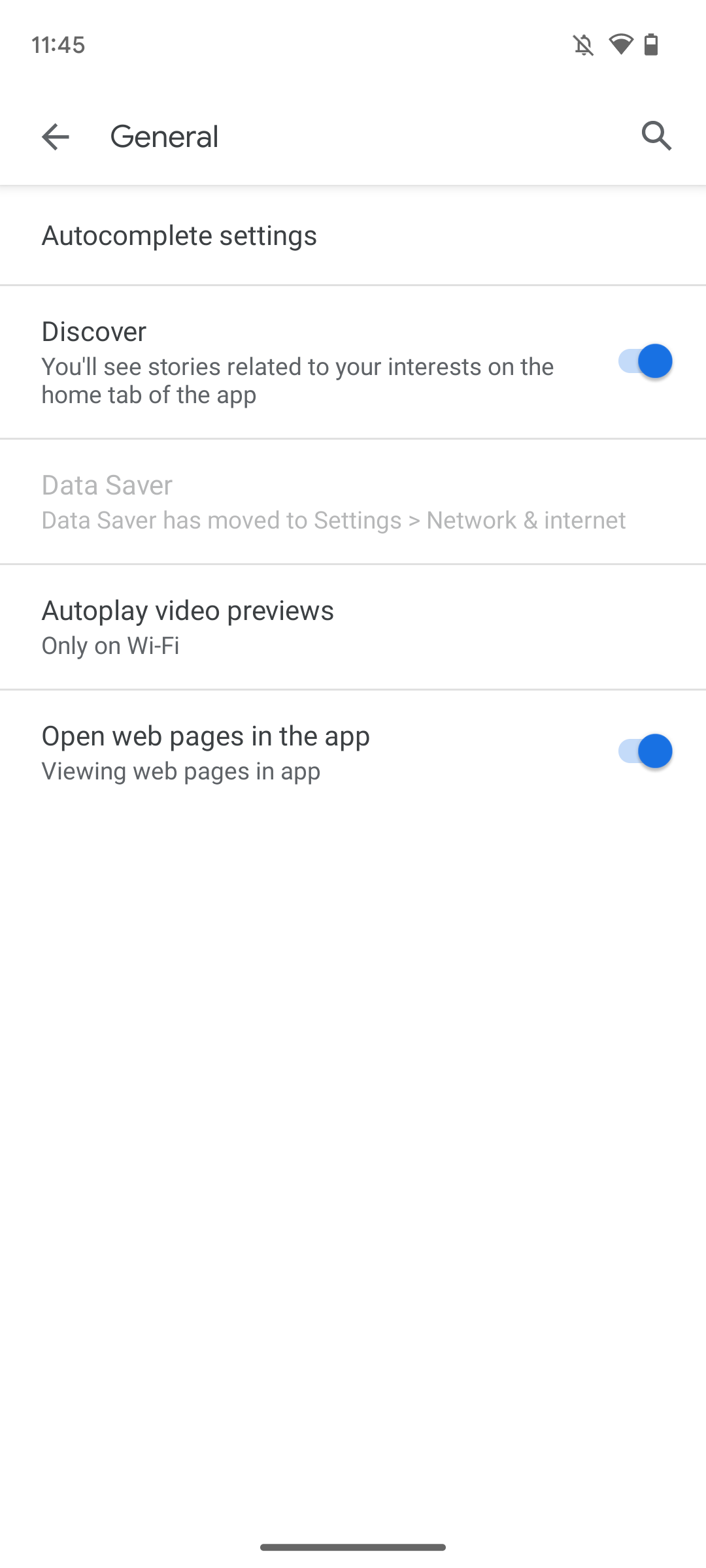This screenshot, captured from a smartphone at 11:45, shows several key interface elements. The phone has approximately half of its signal strength and a battery level at 50%. The top navigation bar includes a 'General' label, with an arrow pointing left on the left side and a search icon on the right. 

The primary section of the screenshot features a white background with various options and settings. A section titled 'Discover' is highlighted, indicating that stories related to the user's interests will appear on the home tab of the app. Another option, 'Data saver,' is printed in light font, suggesting it has either been relocated or disabled; a note beneath it states that 'Data saver' has moved to 'Settings,' under 'Network and Internet.' 

Further down, there is a setting for 'Autoplay of video previews only on Wi-Fi,' and an option labeled 'Open web pages in app,' which includes a prominently enabled blue toggle button, indicating that in-app web page viewing is active.